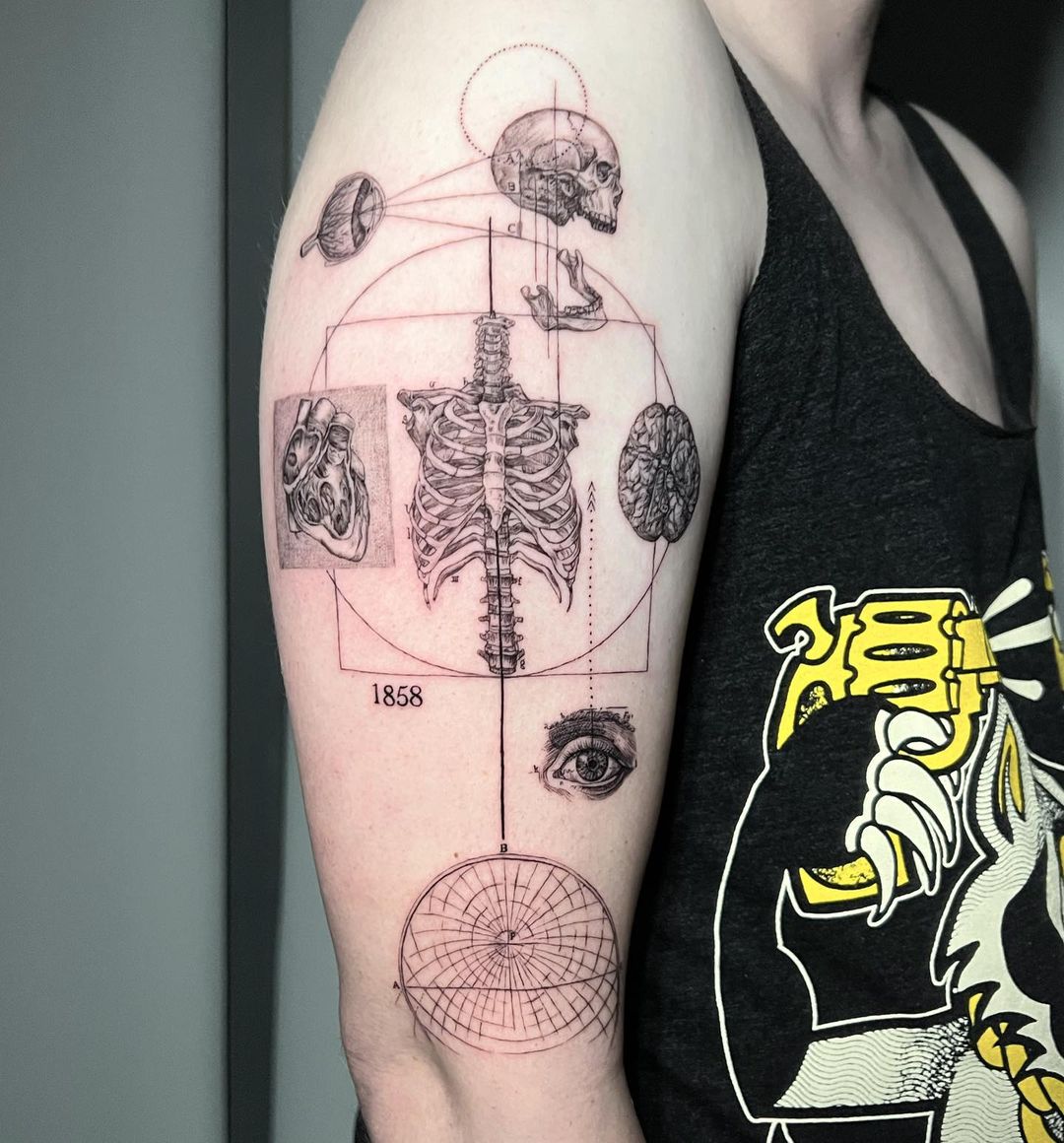This is a highly detailed color photograph of a freshly tattooed arm, starting from the shoulder and ending at the elbow, featuring light-colored skin wearing a black tank top with a yellow and white cartoon character illustration. The tattoo, done entirely in black ink, showcases an elaborate anatomical theme reminiscent of a diagram. The tattoo begins with a side-profile skull at the top, with the detached jawbone positioned just below it. An eyeball is intricately detailed on the upper left, while a rib cage and spine dominate the center, accompanied by a cross-section of a heart and visible arteries. To the right of the rib cage is a top view of a brain, and below it, a detailed depiction of an eye from eyebrow to below the eye. Geometric lines, including a square and circle centered on the rib cage, enhance the visual complexity, leading down to a sphere with concentric circles resembling longitude lines of a globe near the elbow. The number ‘1858’ is inscribed to the lower left of the rib cage. The surrounding redness suggests that the tattoo is quite new and has not yet fully healed.